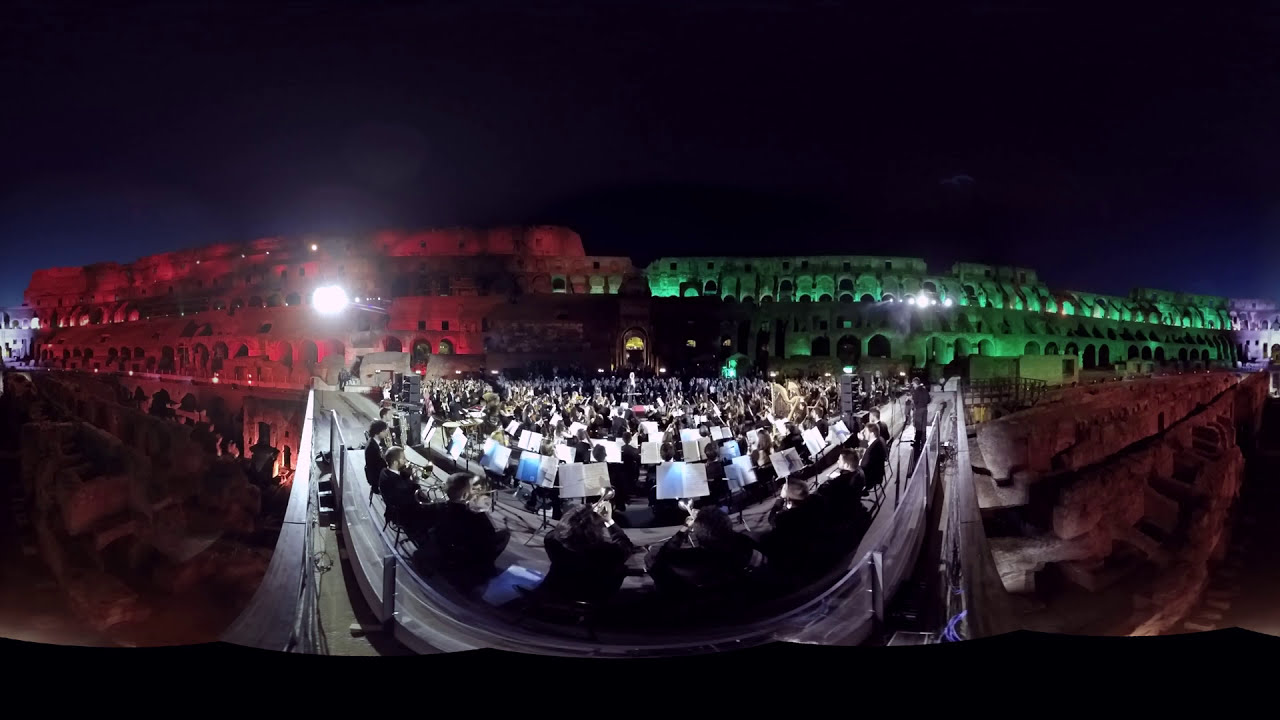The image captures a nighttime outdoor orchestra performance taking place in front of a large, ancient structure resembling the Roman Colosseum. This grand amphitheater is strikingly illuminated, with the left side bathed in a reddish light and the right side adorned in a greenish-white hue. The Colosseum extends across the entire width of the image, forming a dramatic backdrop against the dark night sky.

In the foreground, there is a centrally located stage, slightly lower in the frame, where musicians dressed in black suits are arranged in a semi-circle. They are intently playing their instruments, each with sheet music propped on stands before them. This well-lit stage area contrasts sharply with the darker surroundings, drawing the viewer's attention to the performers. Surrounding the stage, the ambient lighting highlights the ancient and rustic textures of rock figures or structures, framing the central performance.

The combination of the vivid lighting, the detailed historical architecture, and the focused musical performance creates a captivating and immersive visual experience, highlighting the modern utilization of ancient spaces for contemporary cultural events.